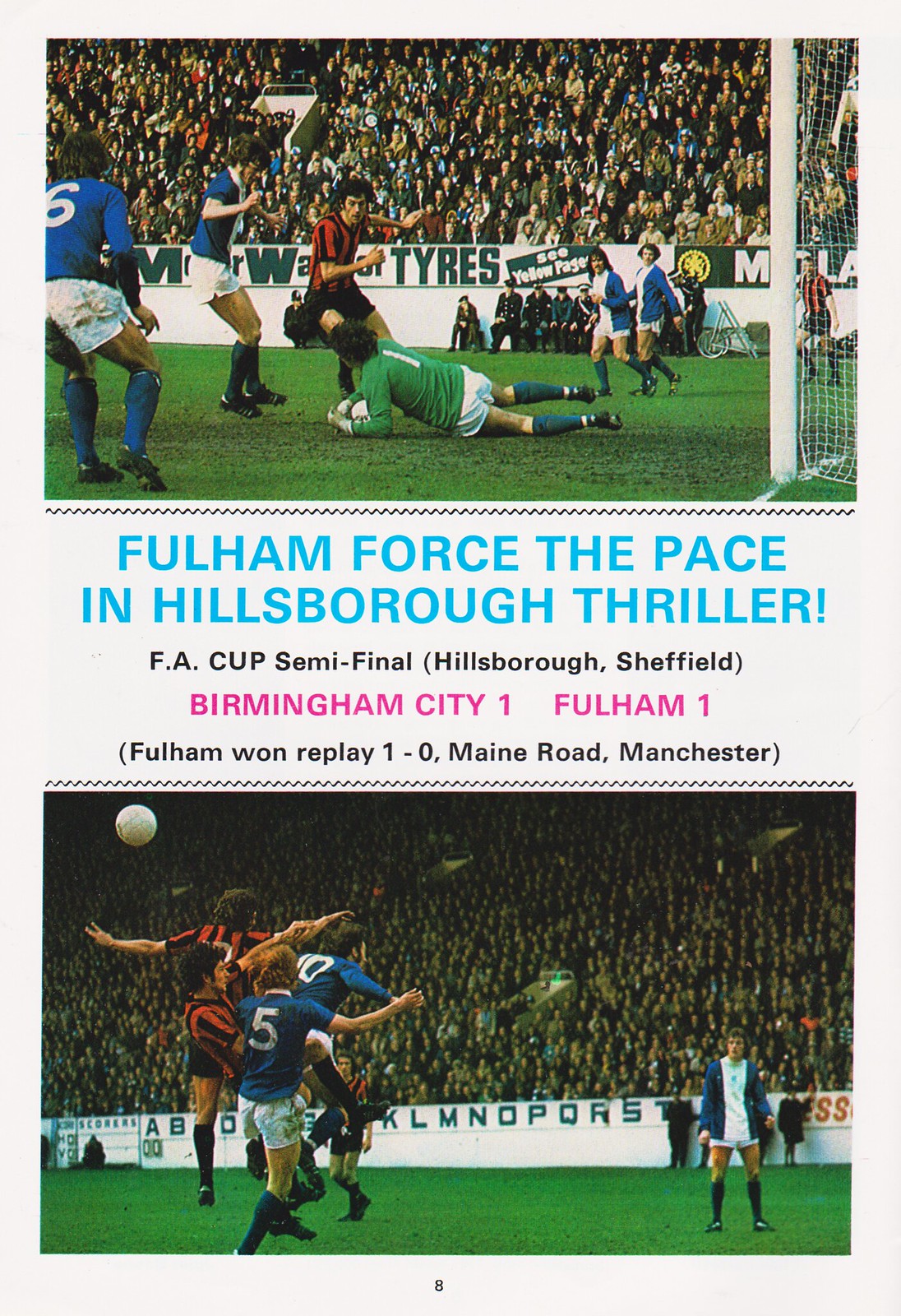This detailed caption provides a comprehensive description of the image, combining key elements from all three interpretations:

"Front page of a match program printed on white cardstock, showcasing a flyer advertising a soccer game. The flyer features two action shots from soccer matches – one at the top and one at the bottom. Both images highlight intense moments on the field against a backdrop of blurry, full stands. In the top image, a goaltender in a green jersey is seen diving to save the ball, surrounded by players in blue kits and red-and-black vertically striped jerseys. The bottom image shows players in blue kits and red-and-black jerseys leaping to head the ball mid-air. Below the top image, in blue font, it reads 'Fulham Force the Pace in Hillsborough Thriller.' Underneath, in black text, the flyer details: 'FA Cup Semi-Final, Hillsborough, Sheffield. Birmingham City 1, Fulham 1.' Beneath that, in purple, it says: 'Fulham 1, Replay 1-0, Main Road, Manchester.' At the very bottom, in small black print, is the number eight."